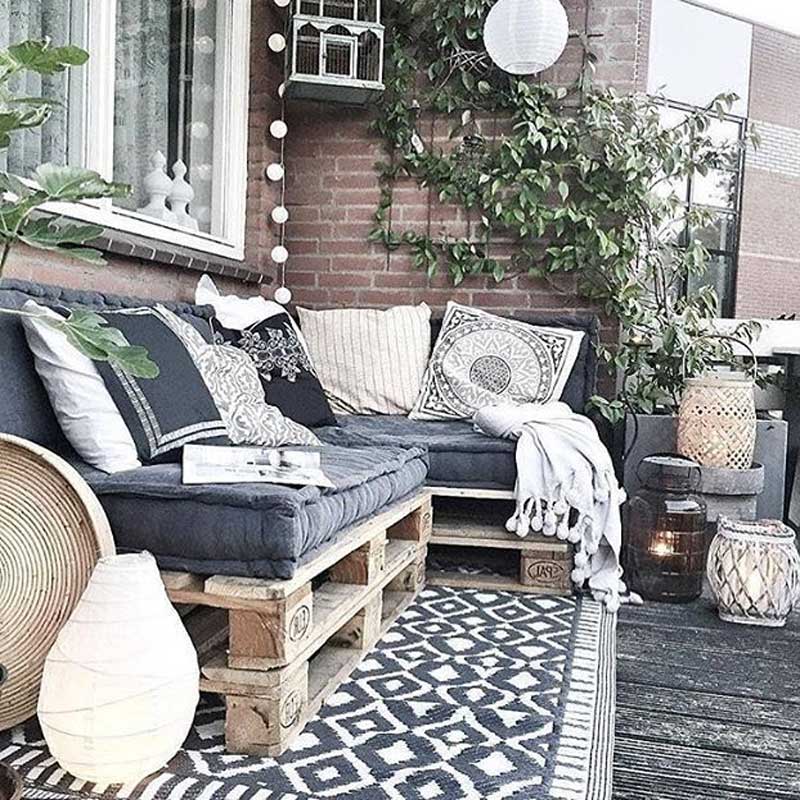This outdoor photograph depicts a cozy seating area on a wooden deck next to a brick house. The focal point is an L-shaped sofa created from stacked wooden pallets, topped with navy blue cushions and accentuated by decorative pillows in navy blue and white, along with a throw blanket. The seating area is situated on a blue and white diamond-patterned rug positioned in the corner where two brick walls meet. An ivy plant climbs up the trellis on the wall facing the deck, adding a touch of greenery. The left-hand wall features a large white-framed window, while the surrounding space is adorned with colorful wicker and ceramic pots. There's also an assortment of decor items, including lanterns and a round wooden tray, enhancing the inviting ambiance of this outdoor retreat.